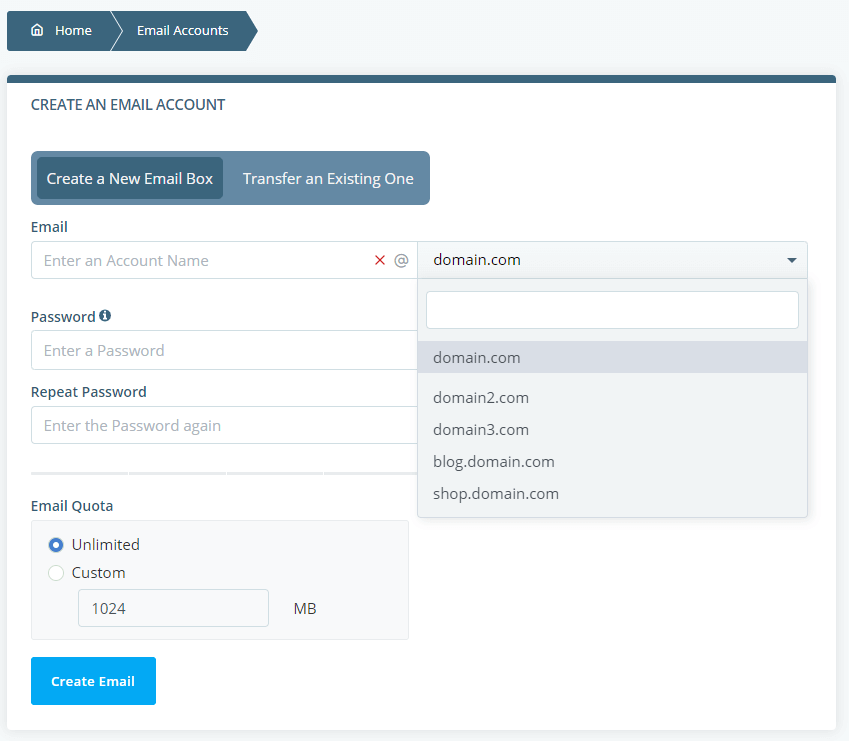The image is a screenshot of an email management interface. At the top, there are navigation options including "Home," "Email Accounts," and a section for creating a new email account. Below this, users can choose between creating a new email mailbox or transferring an existing one. There are fields provided for entering the email account name, selecting the domain from several options such as "domain.com," "domain2.com," "domain3.com," "blog.domain.com," and "shop.domain.com," and setting the password, which needs to be repeated for confirmation. The interface also offers an "Unlimited Email Quota" option and a default setting of "1024 MB" for storage. Finally, a blue button labeled "Create Email" enables users to initiate the creation process. The interface includes a dropdown menu under the "Email Accounts" section, facilitating easy navigation within the system.